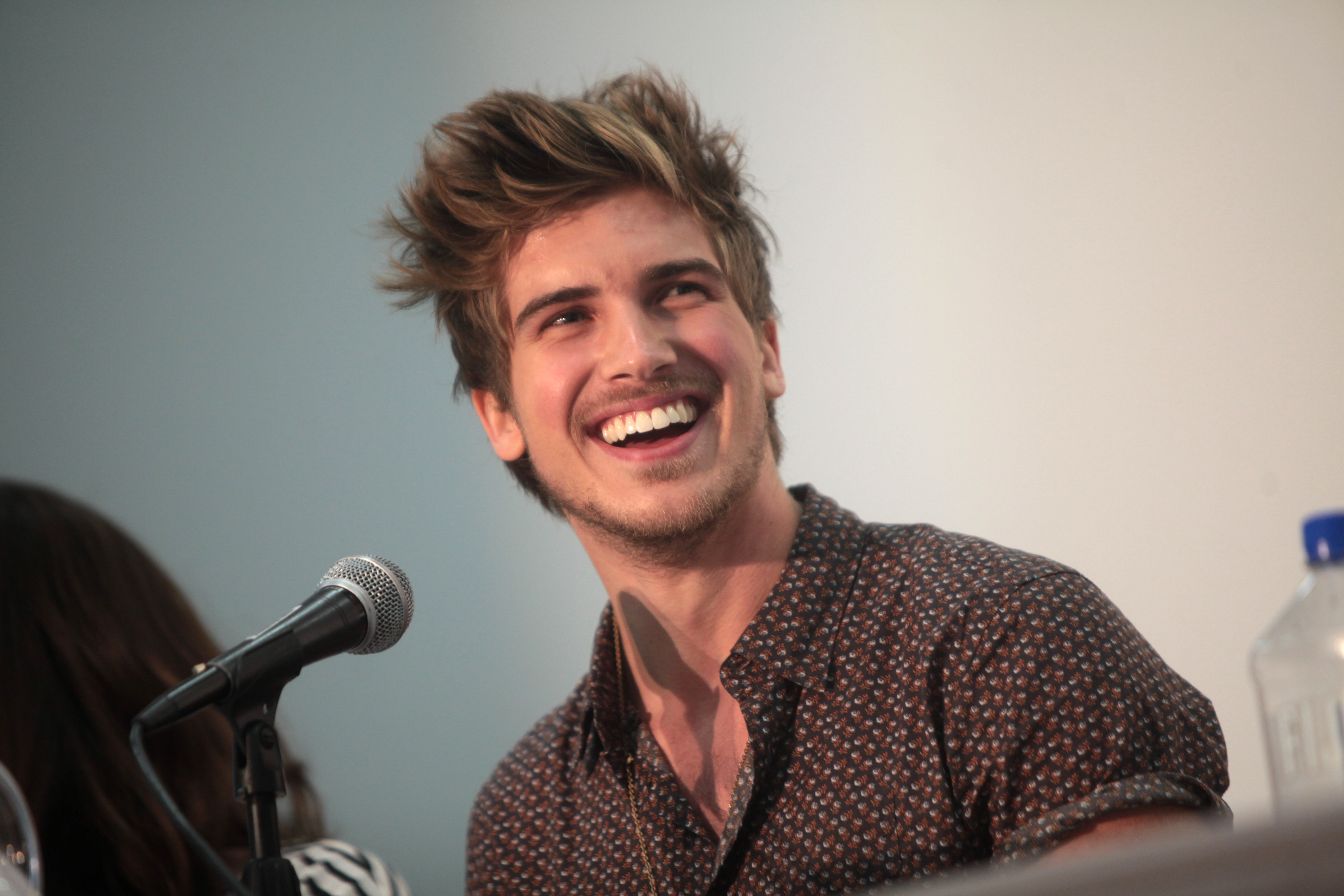The photograph features a young, white man with a broad smile, seated at a table equipped with a microphone stand holding a black microphone with a silver head. His attention is directed slightly upward to his left (the top right of the image). He has medium-length, wild, dirty blonde hair with lighter highlights, styled in an upwards spike, and a bit of beard scruff. He is dressed in a brown collared shirt adorned with red and white polka dots, which is slightly unbuttoned and has the sleeves rolled up above his biceps. A woman with long hair, mostly obscured, is seated next to him. A water bottle with a blue cap is visible at the bottom left. The backdrop of the image transitions from light blue to light beige, giving a distinguished and calm atmosphere. The photograph is wider than it is tall, emphasizing the horizontal layout.